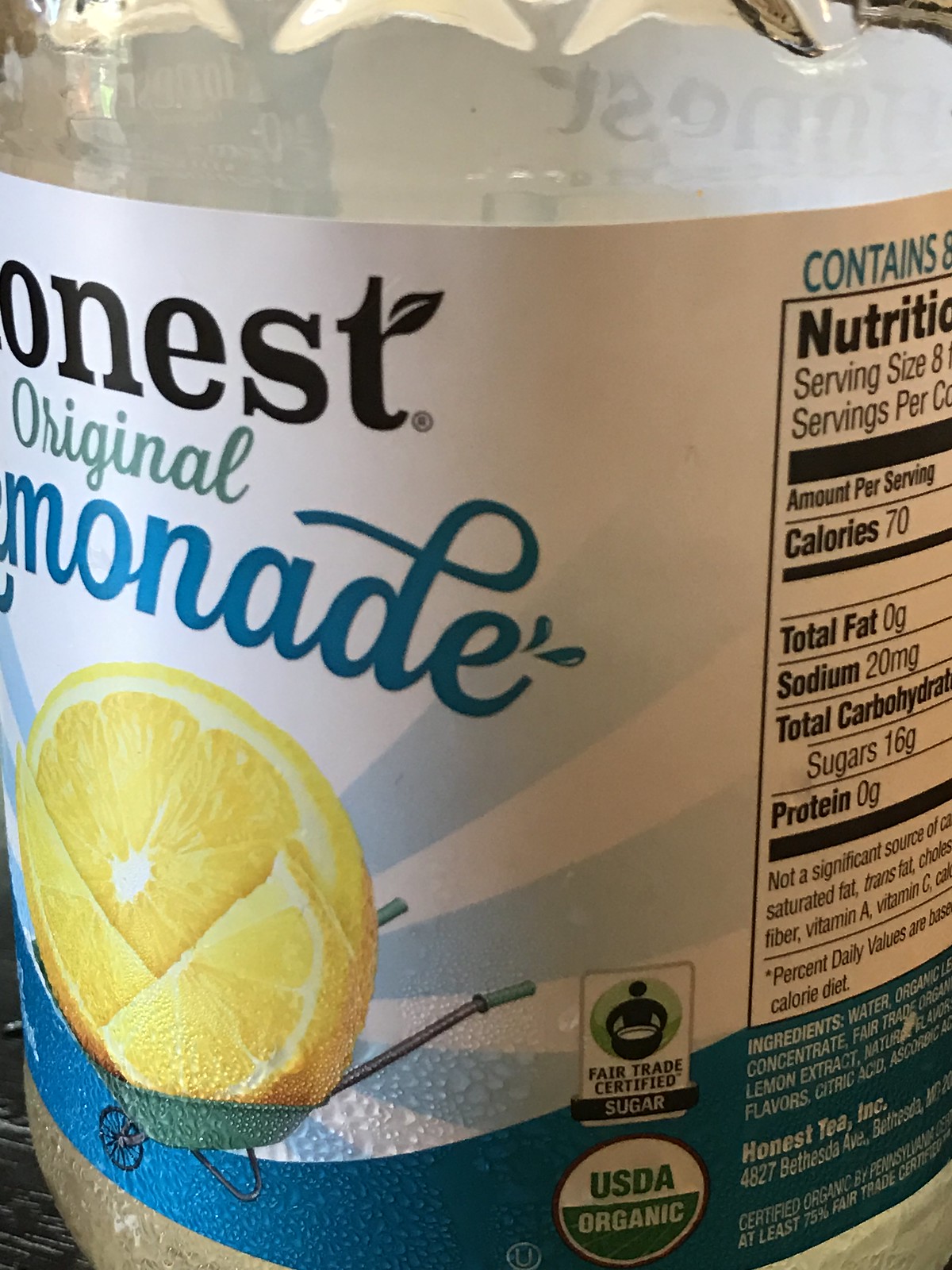This close-up photograph features a bottle of Honest Original Lemonade. The focal point of the image is the front label, which is predominantly white with black, green, and blue text. Central to the label is a vibrant illustration of a large lemon, sliced open, and placed in a green wheelbarrow. The wheelbarrow is brimming with lemon slices, including one whole half and two additional lemon segments. Below the main label, two certification logos are visible: the USDA Organic certification and the Fair Trade Certified Sugar mark. The product is made by Honest Tea Incorporated. The bottle’s nutrition label indicates a serving size of 8 ounces, with each serving containing 70 calories and a notable amount of sugars.